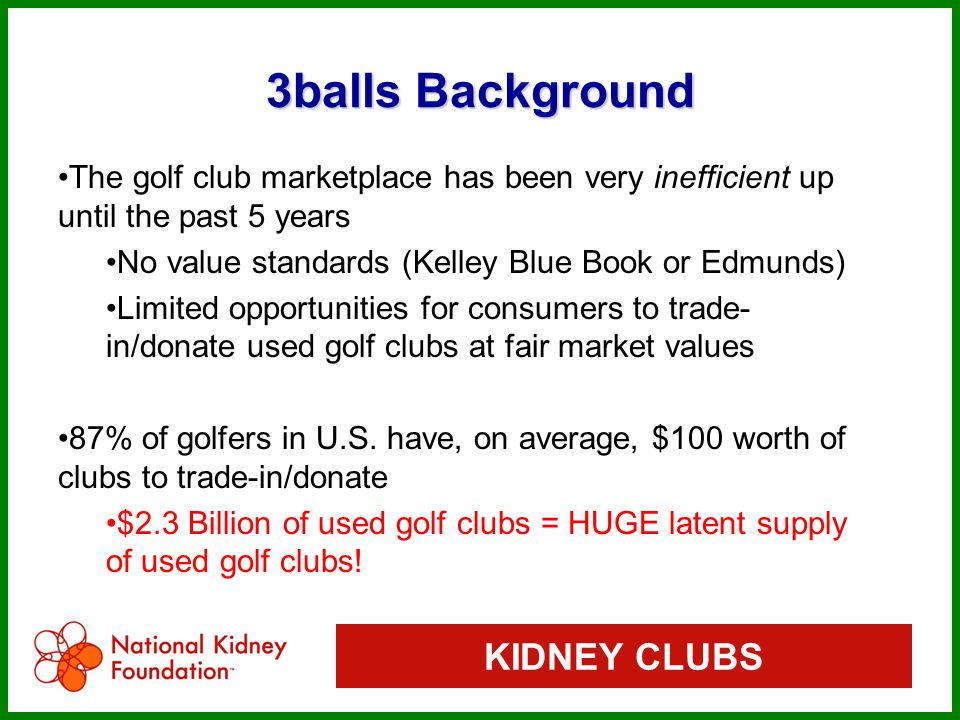The image depicts a PowerPoint slide with a green border, centered around the theme "Three Balls Background," presented in blue text at the top. The slide explores the inefficiency of the golf club marketplace over the past five years. Key bullet points in black text highlight the lack of value standards—such as those provided by Kelly Blue Book or Edmunds—and the limited opportunities for consumers to trade in or donate used golf clubs at fair market values. It notes that 80-87% of golfers in the U.S. possess, on average, $100 worth of clubs eligible for trade-in or donation. Additionally, it states in bold red text that $2.3 billion worth of used golf clubs represents a huge latent supply. The bottom left corner features the National Kidney Foundation’s logo, with the organization's name in red. To the right, a red button with white text reads "Kidney Clubs." The overall design is clear and well-organized.